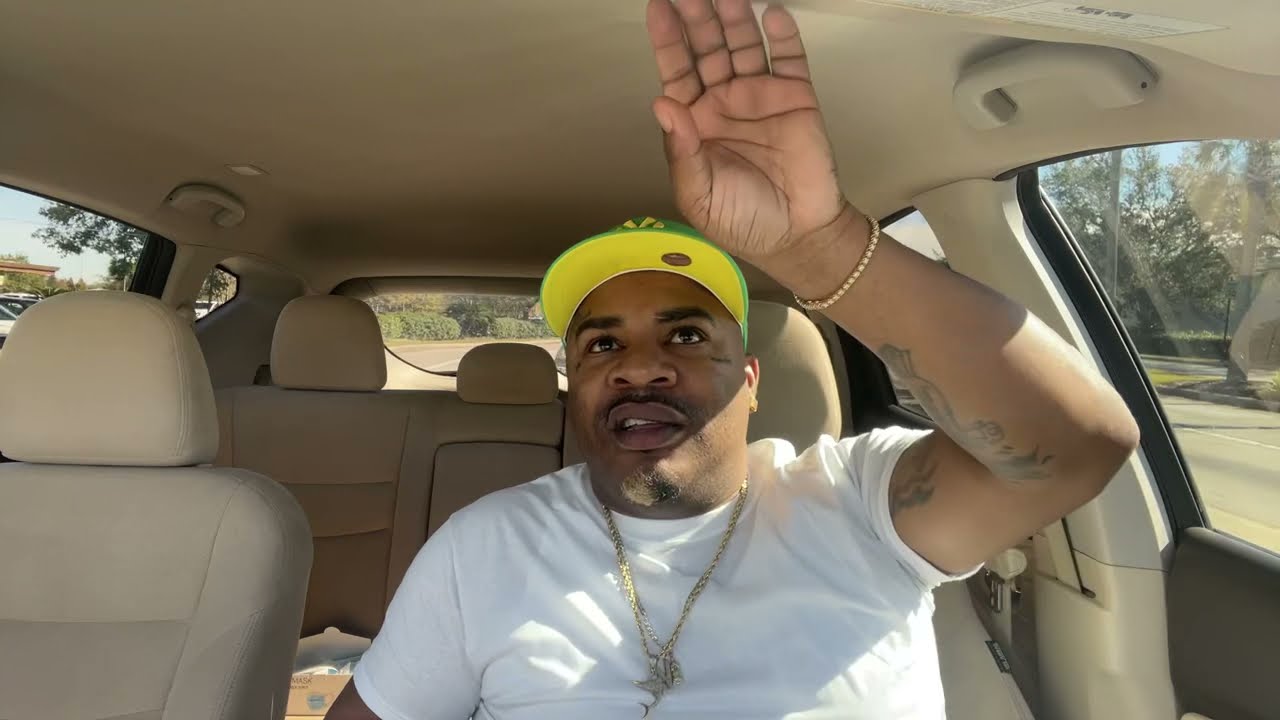In the image, a black man is prominently featured sitting in the driver's seat of a car with a light tan or cream-colored leather interior. He is wearing a green and yellow New York Yankees hat with a visible sticker under the bill. His facial features include a small mustache and a short goatee, along with a tattoo just below his left eye. 

The man is captured mid-motion, reaching up towards the car's visor, revealing a gold bracelet with diamond accents on his wrist and tattoos on his arm. He is dressed in a white short-sleeve shirt with an undershirt visible beneath it. Around his neck, he wears at least two gold necklaces with pendants, one notably shaped like a fish. The car's interior appears clean and well-maintained, with light leather seats suggestive of a luxury vehicle, potentially an SUV.

The background through the car windows indicates a neighborhood setting, and the image has a candid feel, as if it were a snapshot from a live stream or a spontaneous photo taken while driving. The image's colors predominantly feature green, yellow, white, gold, tan, brown, and black, contributing to the overall vividness of the scene.